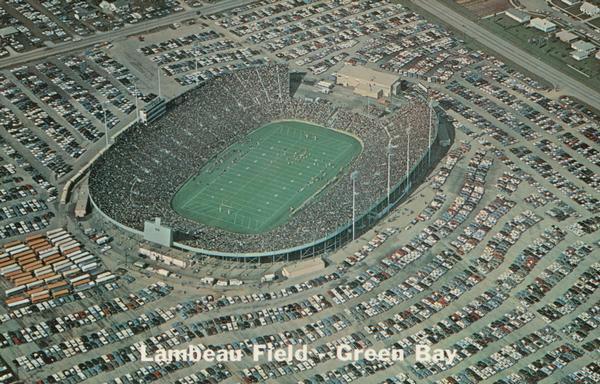This image is an aerial, sepia-toned overhead view of a bustling Lambeau Field in Green Bay. The oval-shaped stadium is situated at the heart of what appears to be a neighborhood, with various seahouses and other buildings surrounding it. The stadium is packed with spectators, indicating a game in progress, although the field is not painted. The relatively small press box is prominent, reflective of an earlier era as suggested by the vintage appearance of the image. The stadium is encircled by a large parking lot filled with thousands of cars, reinforcing the event's significant attendance. At the bottom of the image, "Lambeau Field, Green Bay" is inscribed in white text, further emphasizing the historical and iconic nature of this scene.